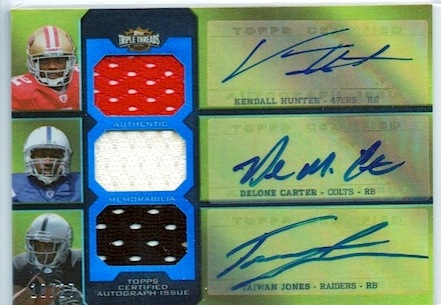This is a detailed graphic of a trading card featuring three American football players, complete with their images, signatures, names, and jersey numbers. The card is slightly wider than it is tall and has a white border, possibly from the plastic wrap it's sealed in. Split into three vertical sections, it prominently displays each player from about the shoulders up, clad in their respective uniforms and helmets.

- On the top left is Kendall Hunter of the San Francisco 49ers, wearing a gold helmet with red and white stripes and a red jersey. Accompanying his image is a red jersey section with white dots. His name and signature are featured on the right side, noting him as a running back (RB).
- In the middle is Delone Carter of the Indianapolis Colts, depicted in a white helmet with a blue stripe and a blue jersey. To the right of his image is a piece of his white jersey. His name and signature are displayed alongside, identifying him also as a running back.
- The bottom position is occupied by Taiwan Jones of the Raiders, wearing a silver helmet with a black stripe and a black jersey. A piece of his black jersey with white dots is shown. His name and signature are positioned on the right, designating him as a running back.

The background pattern features a sequence of octagonal shapes in red, white, and black, adorned with dots. At the very bottom, in small white lettering, the card reads, "TOPS Certified Autograph Issue," indicating its status as an authenticated collectible. The main colors of the design include black, white, red, blue, and green, contributing to its vibrant and visually striking appearance.